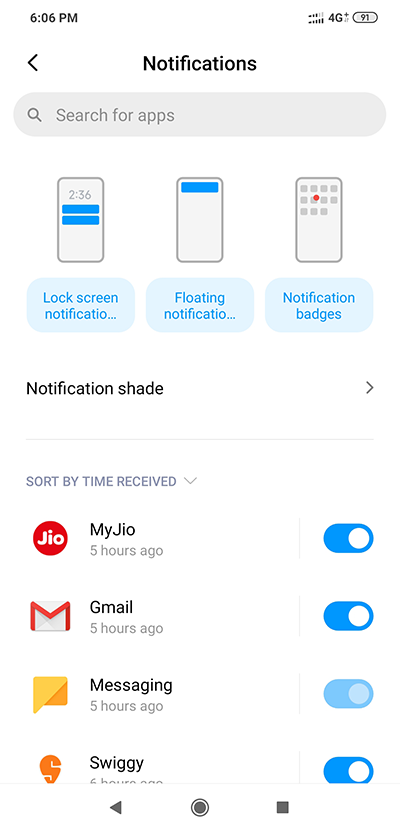The image displays a smartphone screen with the current time shown as 6:06 PM at the top left corner, alongside a signal indicator showing a 4G connection and a battery level at 91% on the top right. Below this status bar, the screen displays the notification panel. Immediately beneath the status bar is a grey search dialog for searching apps.

The main content of the notification screen features three miniature images of a smartphone, each illustrating different notification settings:
1. The first image, titled "Lock Screen Notifications," shows blue bars approximately in the center of the screen.
2. The second image, labeled "Floating Notifications," displays a blue bar at the top of the screen.
3. The third image depicts a grid of app icons with one app marked by a small red dot, under the heading "Notification Badges."

Below these visuals, there is a section titled "Notification Shade" accompanied by an expandable menu icon on the right. In this section, a list of apps is displayed, each with its notification status:
- MyGeo: Enabled
- Gmail: Enabled
- Messaging: Not Enabled
- Swiggy: Enabled

The detailed layout suggests the user is customizing or reviewing notification settings for various apps on their smartphone.